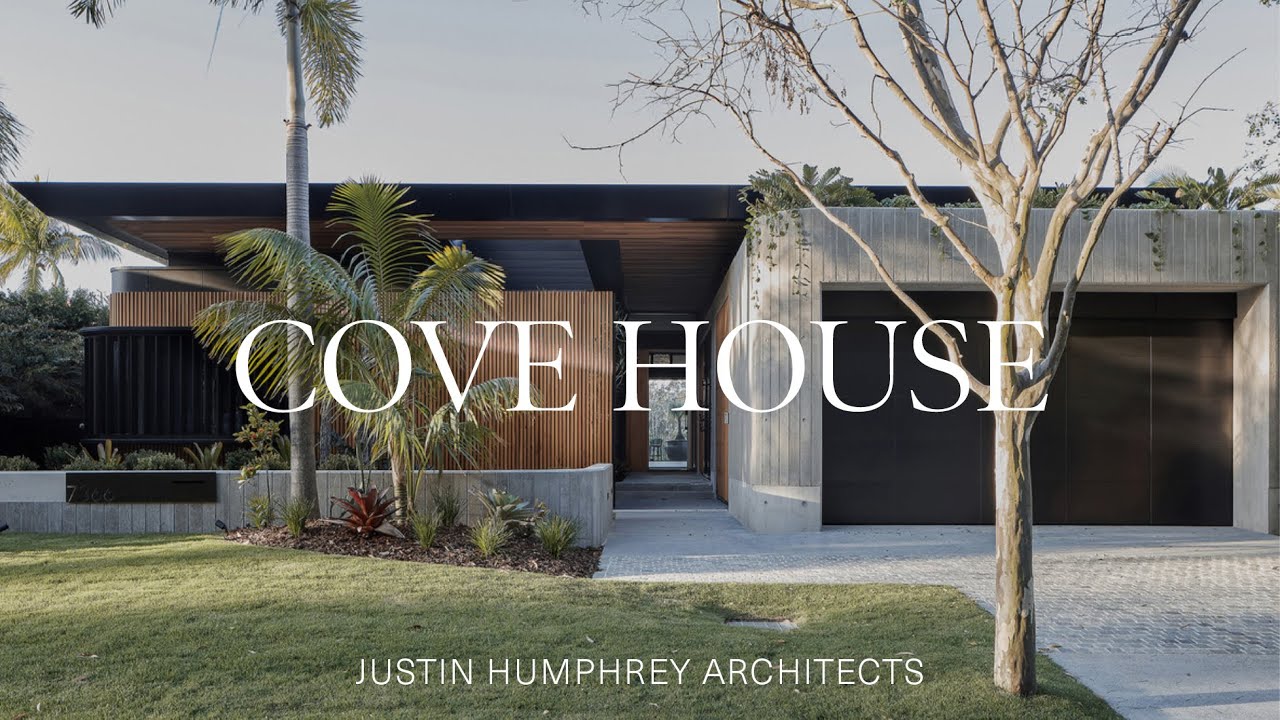The image is a high-resolution photograph of an elegant, modern house featured in an architectural advertisement. The house showcases a sophisticated design attributed to Justin Humphrey Architects, indicated by text at the bottom in small, all-caps white font. The central caption reads "COVE HOUSE" in prominent all-caps white font.

On the right, the structure features a distinct garage with an exterior lined in rows of wood stained to mimic concrete, giving it a gray, almost industrial appearance. The garage door is a dark brownish-black hue. Above the garage, lush greenery cascades down in the form of vines, adding a touch of nature to the sleek design. 

The left side of the house presents a different aesthetic with a façade constructed of bamboo-like wooden slats and complemented by a modern, flat black roof, exuding a minimalist, almost Japanese-inspired feel. A black railing and thin wooden slats, likely bamboo, frame the porch area. The interior glimpses show a warm brownish tint, contributing to the home’s squat and spacious ambiance.

Adding to the home's charm are palm trees, other green vegetation, and a meticulously maintained lawn. A small tree is positioned on the left-hand side of the brick driveway and walkway, contributing to the overall picturesque and serene outdoor setting. The setting is captured on an overcast day, enhancing the tranquil and inviting atmosphere of this modern architectural marvel.